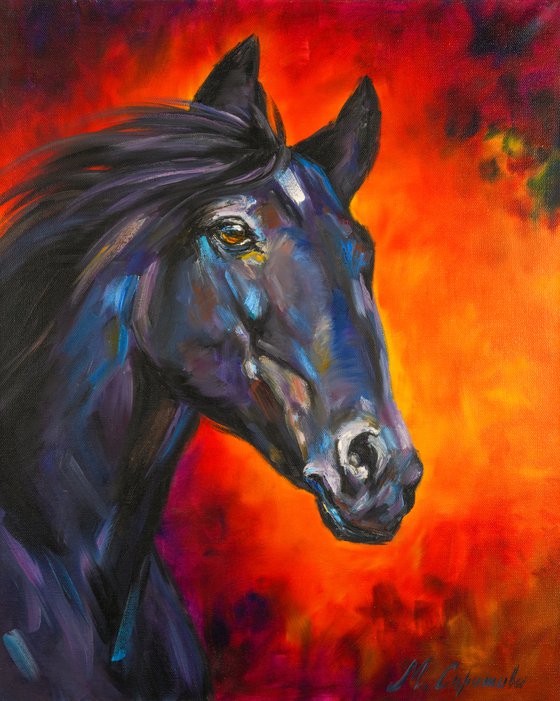The painting showcases a powerful and majestic black horse, its profile accentuated by a fiery backdrop that gives the impression of a blaze raging behind it. The horse’s coat, though primarily dark, is brought to life with intricate highlights of blue and purple that suggest the interplay of light and shadow, adding depth and dimension to its form. The ears are erect, and the soulful brown eyes gaze forward, imbuing the horse with a lifelike presence despite the artwork's stylized approach. The artist has effectively used non-photorealistic techniques to convey the essence of the horse, focusing on the neck and upper shoulders. The dramatic background, which resembles an intense fire, further emphasizes the dynamism and vigor of the subject. This visually captivating piece is signed in the lower right corner by M. Caramole, cementing the artist’s touch on the beautiful representation.